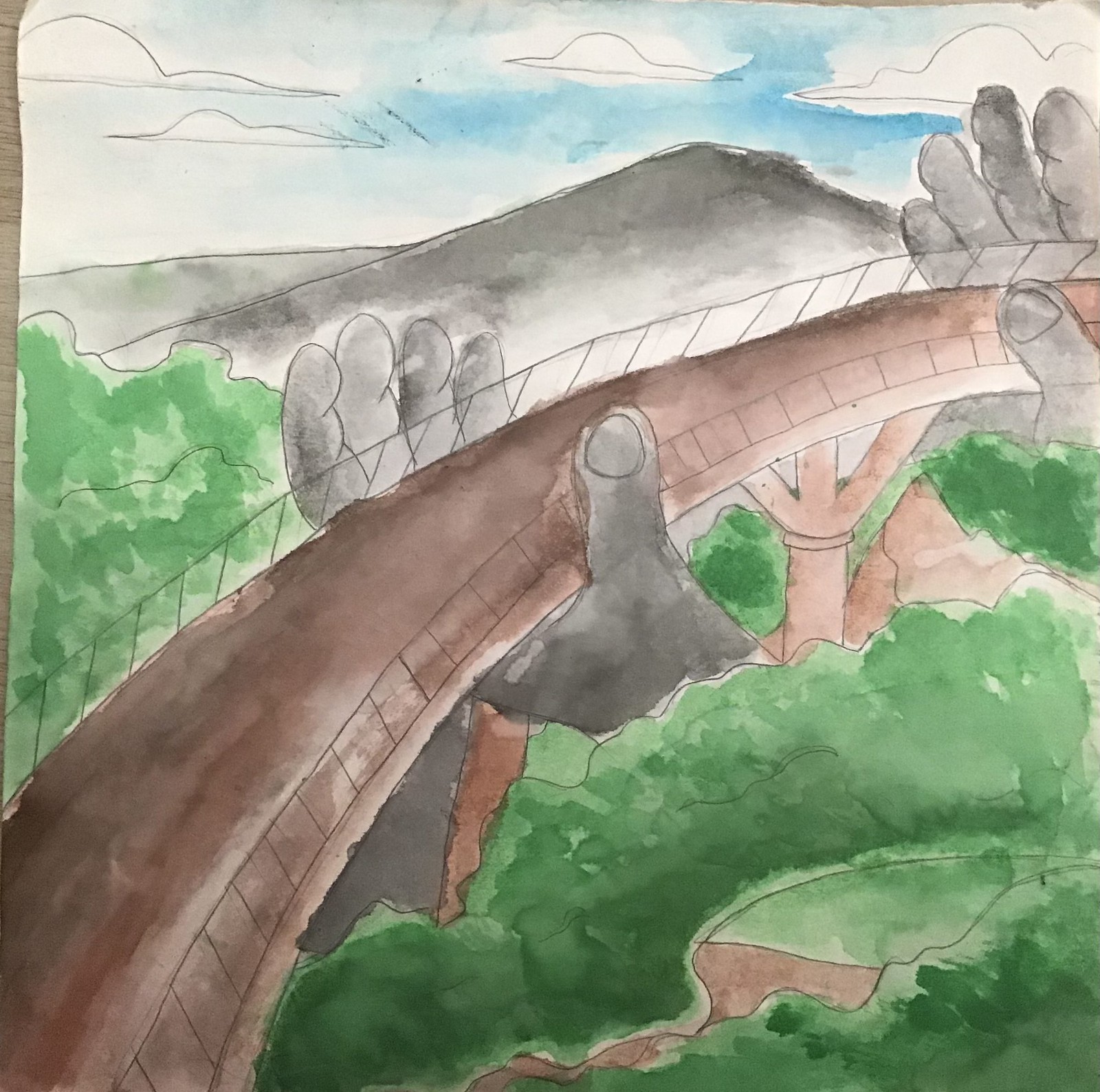The watercolor painting features a tranquil scene dominated by a vibrant robin egg blue sky adorned with fluffy white clouds. In the background, a mountain shaded in hues of gray and black stretches across, providing a majestic backdrop. Below, a substantial brown bridge with a guardrail extends diagonally from the lower left corner through the center, finally trailing off towards the right. This bridge is uniquely supported by two large hands, shaded in black and gray, adding an intriguing focal point to the painting. The landscape around and beneath the bridge is lush with greenery, depicting treetops, bushes, and possibly a river or stream that subtly blends shades of green and pink. The overall composition, with its mix of natural and surreal elements, creates a visually captivating and serene scene.